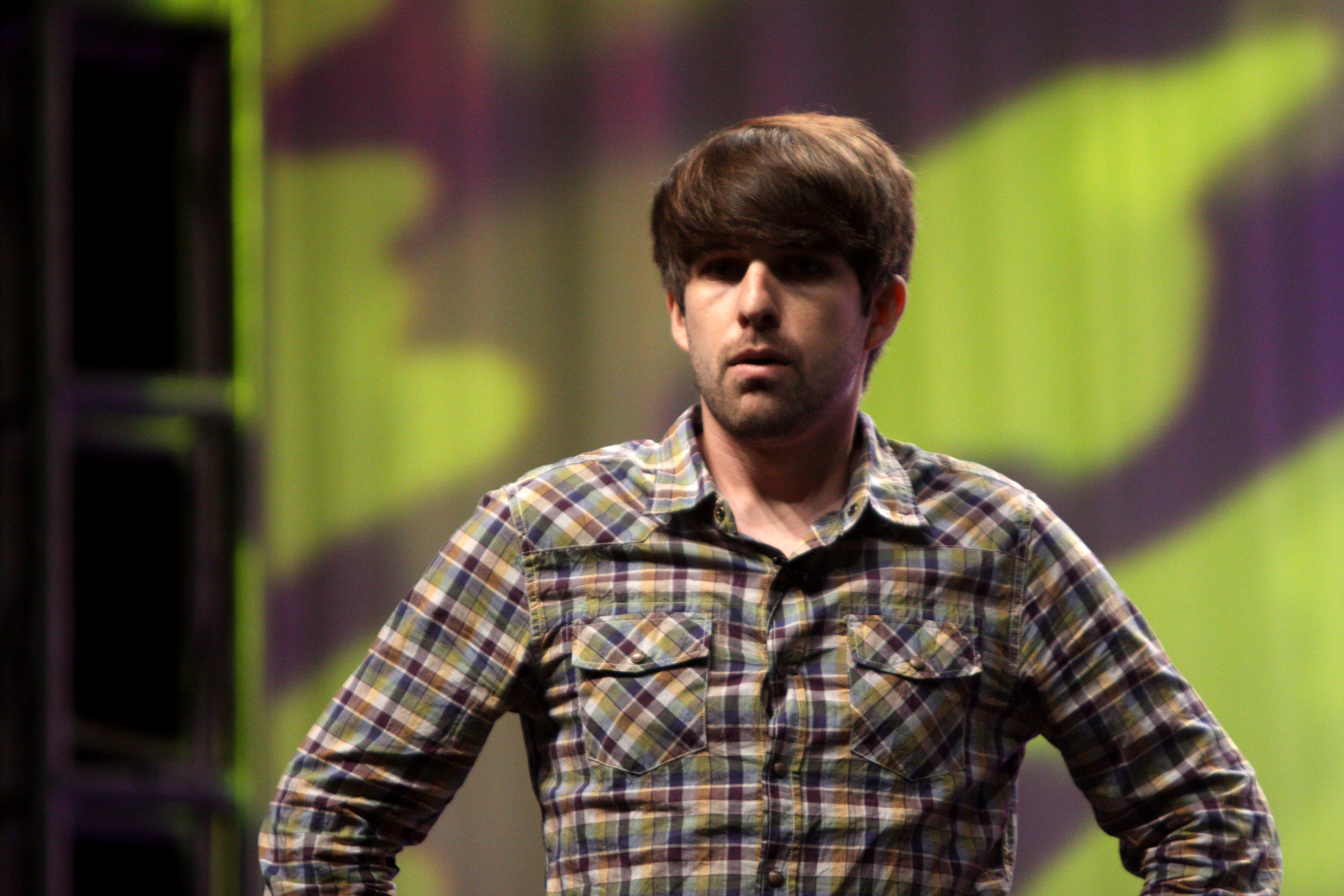This photograph features a man, likely a white male, viewed from the ribcage up. He has dark brown, thick shaggy hair, styled so that his side-swept bangs reach his eyebrows, partially shadowing his eyes. His face is adorned with a dark brown beard and mustache. He is wearing a green, white, blue, and black plaid button-down collared shirt, which is notably wrinkled, with two chest pockets that have flap buttons. His elbows are bent, suggesting his hands are on his hips. The background is out of focus, featuring a long, large green and purple curtain with black designs and pleats. Additionally, there appears to be a metal structure to the left, through which black and other indistinct shapes are visible.